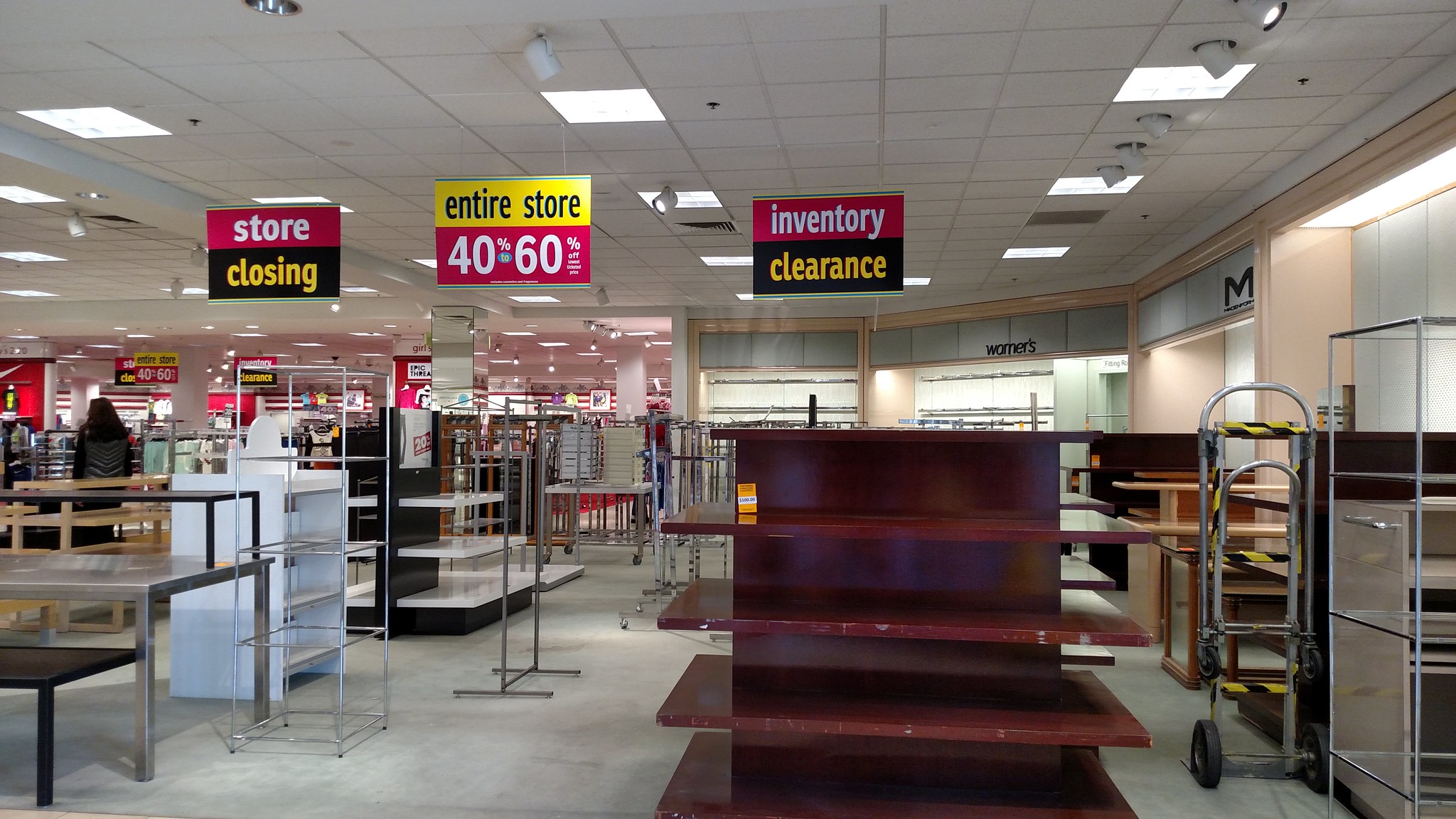Inside a brightly lit retail store, the ceiling is lined with pristine white tiles and features a mix of built-in square fluorescent lights, canister lights, and spotlights hanging down. Brightly colored signs in yellow, red, and black hang from the ceiling, announcing "Store Closing, Inventory Clearance" and "Entire Store 40-60% Off." The store's atmosphere reflects the final stages of a clearance sale, with barren walls that once labeled "Women's" and "Men’s" sections now stripped of signage. Shelves are largely empty, and a few dollies are scattered about, emphasizing the sparse inventory and the imminent closure.